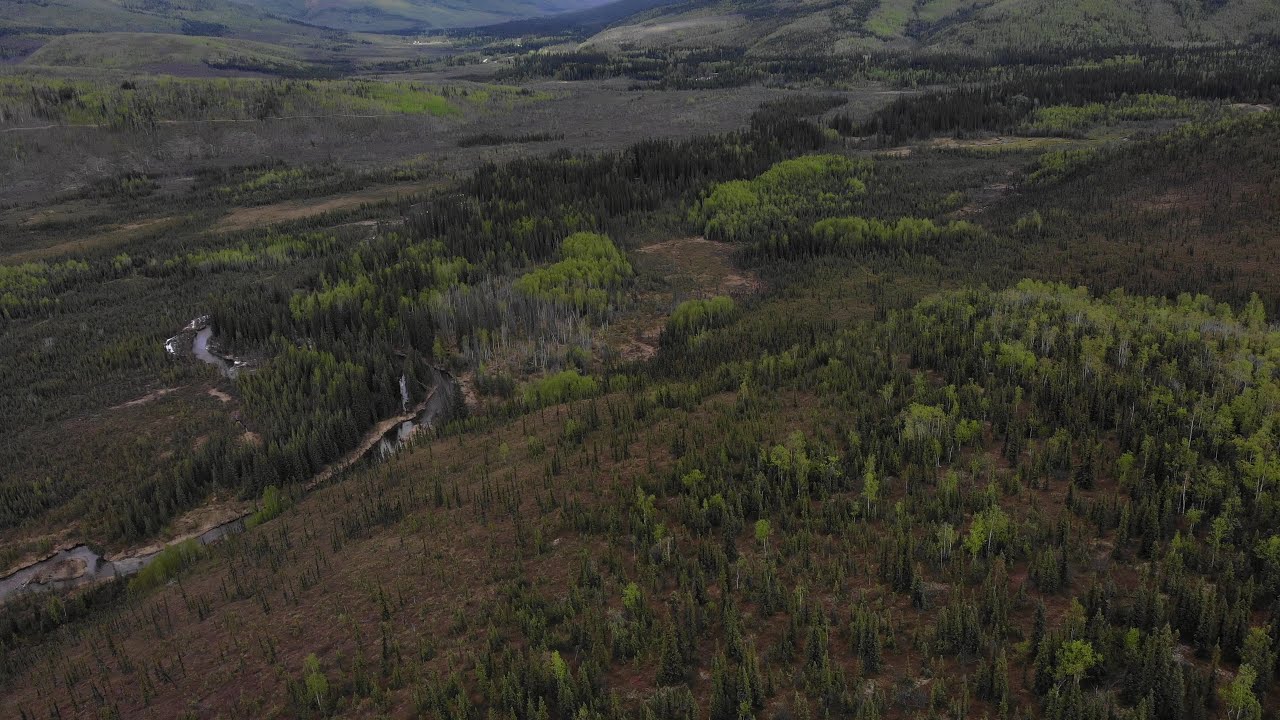The photograph showcases an expansive landscape of hills and valleys, captured from an elevated vantage point, offering an almost aerial perspective. On the right side of the image, a prominent hill is visible, its brown ground interspersed with patches of green grass and clusters of trees. The trees vary in color, ranging from dark green to light green, with some dry trees scattered throughout. To the left, a lush valley filled with similar vegetation extends into the distance, where more hills and valleys continue the undulating terrain. A winding road or possibly a body of water cuts through the valley, adding a sense of depth and movement to the scene. The overall color palette of the photograph is dominated by earthy browns and rich greens, with subtle touches of reddish hues and a sliver of blue sky peeking at the top, indicating it was taken during the daytime. The clear, natural light enhances the vivid details of the terrain, while no people, animals, or homes are visible, emphasizing the untouched and serene nature of the landscape.